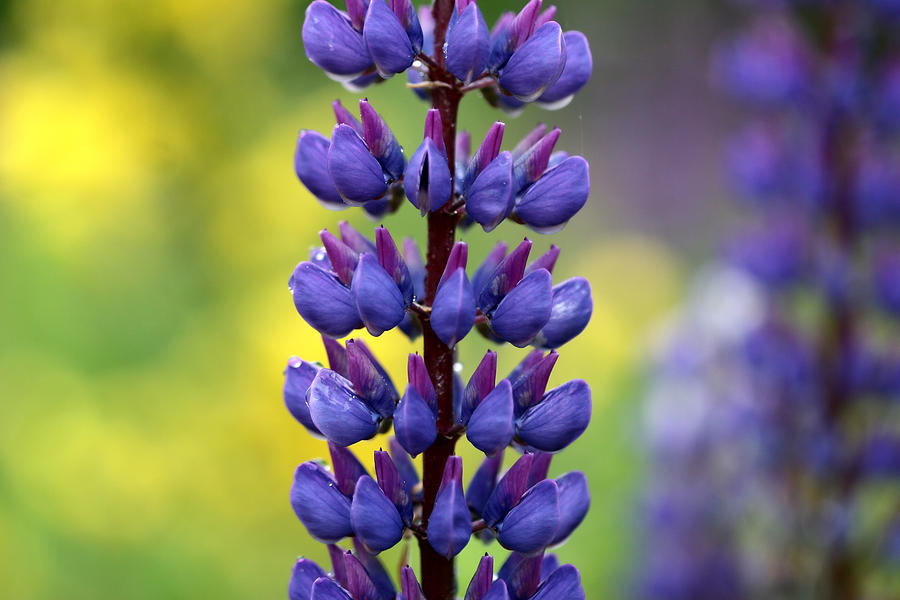This photograph depicts a vivid close-up of a cylindrical stem of a flower, running vertically through the center of a horizontal frame. The stem, a thick, reddish-brown maroon, is adorned with six distinct circular tiers of intricate clamshell-shaped flowers. These flowers, varying in shades of blue, purple, and violet, boast dark blue veins and intricate patterns on their petals. Each tier showcases delicate, clam-like blooms, primarily closed, with one near the top slightly open. The uppermost row features eight flowers, mirrored by the next row below, with the third row containing nine flowers. The background, rich with blurred details, shows a similar flower out of focus on the right side of the frame, amidst a greenish-yellow blur suggestive of grass and foliage. The overall image emphasizes the sharp, captivating beauty of the central flower against a softly obscured garden backdrop.